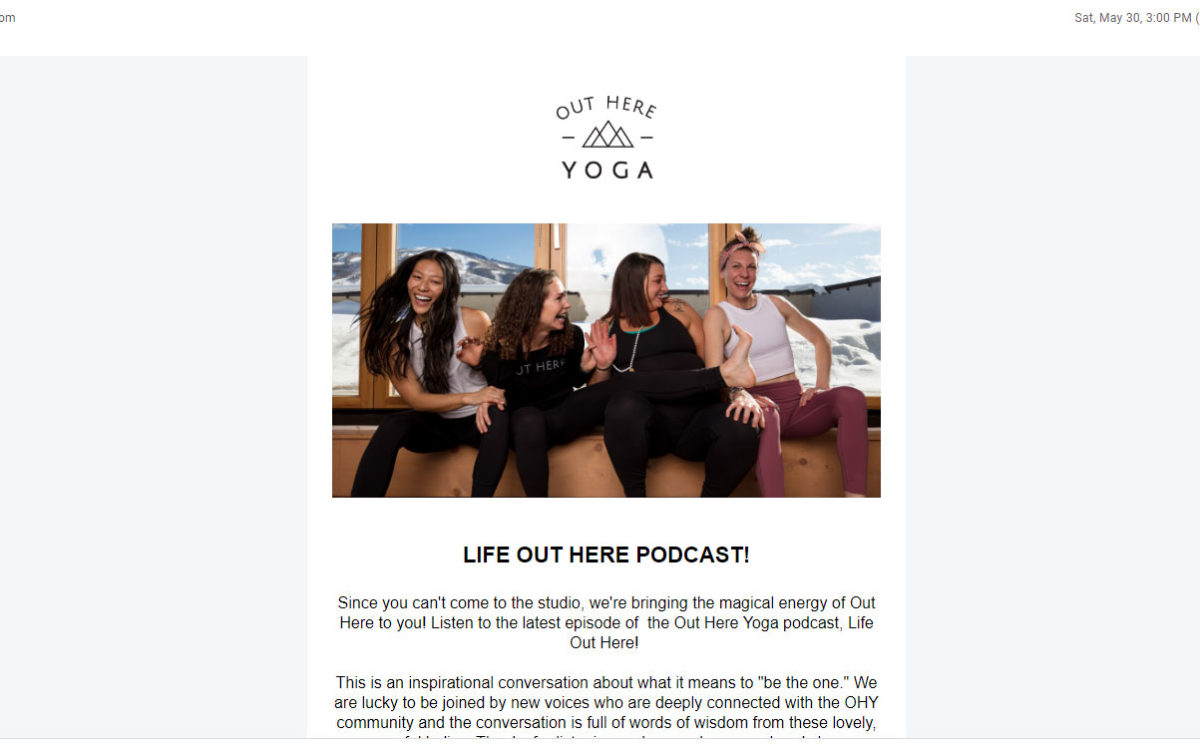The image depicts a screenshot likely taken from an email associated with a yoga website or platform. This screenshot serves as a flyer, featuring a primarily dark gray or light gray background with a content block centered in the middle. The edges of the image provide clues to its origins, as the top left corner displays a truncated part of an email address ending in ".com," aiding in identifying it as an email. The right-hand side marks the date and time when the email was sent: Saturday, May 30th, at 3 p.m.

At the top center of the flyer, the text "Out Here Yoga" is prominently featured. Positioned between "Out Here" and "Yoga" is a symbol depicting a mountain flanked by two dashes. Just below this heading, a cover banner stretches across the page, showcasing an engaging image of four women. These women, dressed in workout attire, are seated against a backdrop of wooden doors with adjoining windows. The windows reveal a scenic view of dark, snow-capped mountains. The women appear to be enjoying a moment of camaraderie, laughing and acting playful.

Directly beneath this banner image, a bolded subtitle reads "Life Out Here Podcast." Following this subtitle is a concise description presented in two paragraphs. This description provides insightful details about the podcast, informing recipients about its content and relevance to the audience.